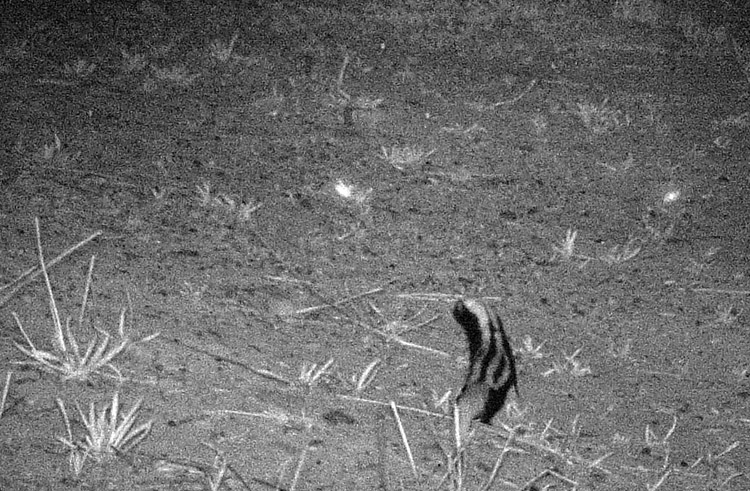The image appears to be a blurry, grayscale or night vision photograph, likely taken with a wildlife camera often used by scientists. It captures a barren, rough terrain landscape with patches of dried grass and sparse shrubbery. The focal point of the image is near the center, possibly in the lower right quadrant, where a small black and white creature, presumed to be a skunk, is visible. This animal features distinctive white stripes along its black body and may have a white tail. The scene suggests the skunk might be walking upright, though the image's poor quality makes it difficult to discern specific details. Additionally, there are two beams of light above the creature, possibly from a car's headlights reflected in the camera.